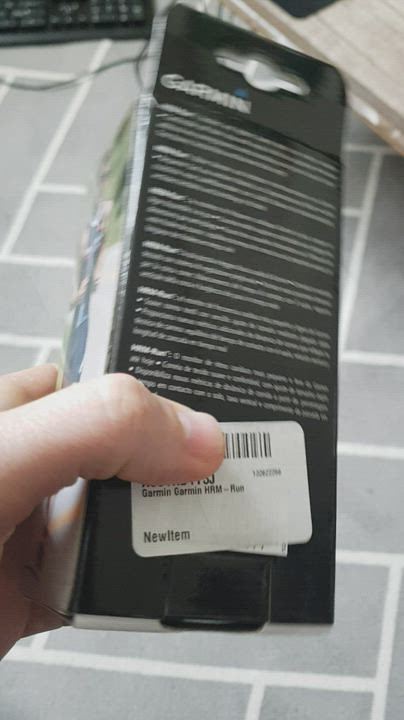A close-up photograph captures a rectangular product package held by a male, Caucasian hand. The brand name "Garmin" is visible at the top of the package, though the fine print and exact details on the back are blurred and difficult to decipher. The person's thumb partially obscures a barcode and a label on the package. An annotation indicating "new item" is also discernible amidst the blurry text. The background features a gray and white brick pattern, likely on a tablecloth.